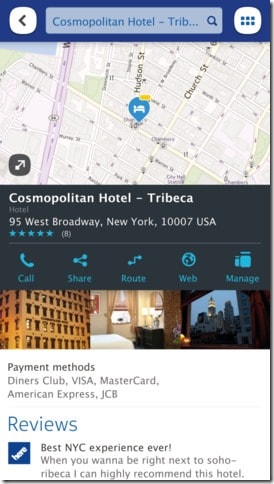Screenshot of a Website on a Mobile Device: Detailed Description

The image is a screenshot of a website, likely viewed on a mobile device. Central to the image is a grayish-colored background, indicating the color scheme of the website. At the top middle, a rectangular-shaped address bar displays a partial URL in blue text: "Cosmopolitan Hotel - T-R-I-B...". This hints that the website pertains to the Cosmopolitan Hotel, located in the Tribeca area.

In the top left corner, there is a distinct, square-shaped logo with rounded edges, featuring a black arrow pointing to the left, set against a white background. The top right corner mirrors this shape but contains six small blue squares arranged in a grid.

Dominating the middle portion of the image is a map of a city, presumably New York, based on the adjacent text. Below the map, white text reads: "Cosmopolitan Hotel, Tribeca, Hotel, 95 West Broadway, New York 10007 USA," clearly indicating the hotel's location.

The lower half of the image displays several navigation options in highly saturated blue text, which include "Call," "Share," "Route," "Web," and "Manage." Beneath these options, a photo of a hotel room is visible, showcasing a comfortable bed, a nightstand, and a partial view of the city outside the window.

At the very bottom of the image, blue text labeled "Reviews" can be seen, followed by a review snippet stating, "Best New York experience ever."